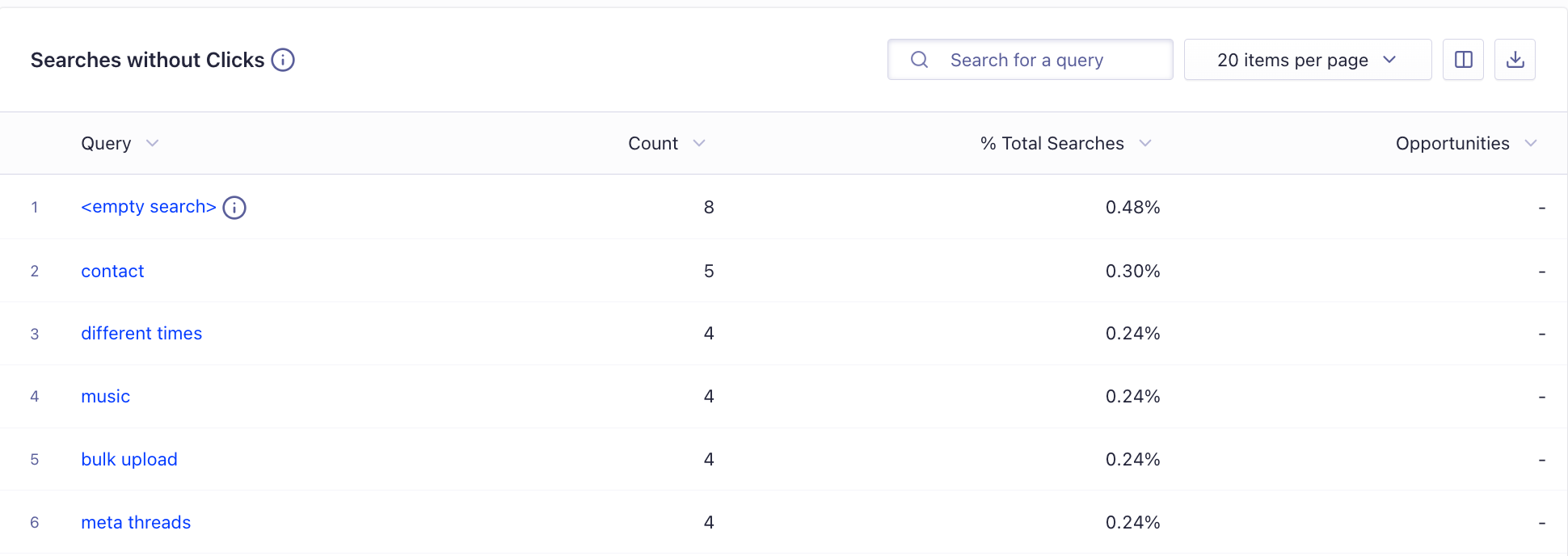This page displays a text-based summary of search results that yielded no clicks. At the top, a search box for entering query terms and a drop-down menu are available, with the option to show 20 items per page by default.

Beneath the heading "Searches Without Clicks," six specific queries are listed, each accompanied by their respective counts and percentages of total searches:

1. **Empty Search**: Count of 8, making up 0.48% of total searches.
2. **Contact**: Count of 5, comprising 0.30% of total searches.
3. **Different Times**: Count of 4, representing 0.24% of total searches.
4. **Music**: Count of 4, contributing to 0.24% of total searches.
5. **Bulk Upload**: Count of 4, equating to 0.24% of total searches.
6. **Meta Threads**: Count of 4, also making up 0.24% of total searches.

Each query is organized in descending order based on the number of searches without clicks, highlighting search trends and potential areas for content improvement or user experience enhancements.